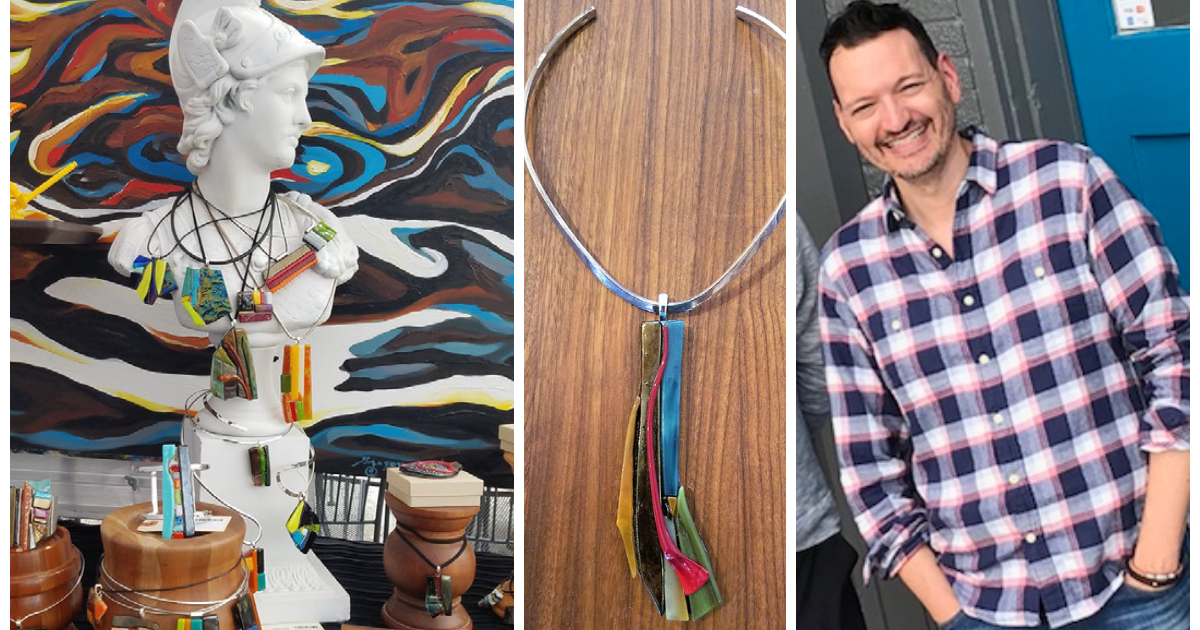The image is a triptych of three distinct yet related photographs, all in vibrant color. The leftmost picture features a white marble statue that resembles a Greek god, adorned with an assortment of eclectic handmade necklaces, each crafted from an array of materials strung on black wire. This statue is set against a dynamic backdrop with wave-like patterns. The central photograph spotlights one of these unique necklaces. It is a sterling silver choker, open at the back, with various multicolored materials hanging in a three-inch grouping from its center. Finally, the rightmost image captures the artist, a man with short dark hair, stubble, and a mustache. He is smiling warmly, squinting slightly, and leaning to the left. Clad in a pink, white, and purple plaid flannel shirt with white buttons and his hands in the pockets of his jeans, he exudes a sense of contentment. His casual pose suggests a friendly and approachable demeanor, which complements the artistic flair exhibited in his jewelry. This series highlights both the artist and his distinctive, colorful creations.